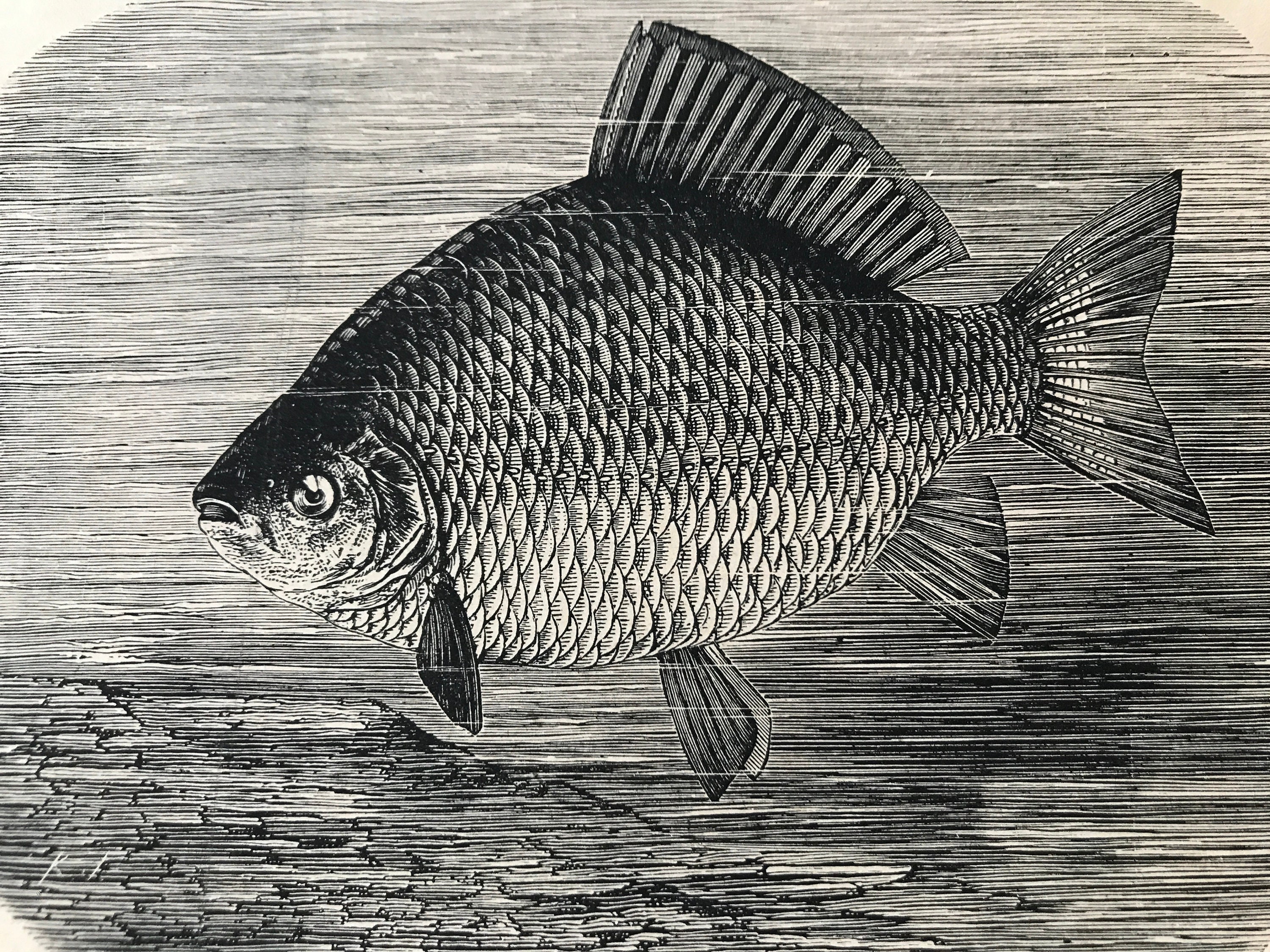The image is an intricate black ink line drawing of a fish with a disc teardrop-shaped body. The fish is oriented facing the left side of the image and is prominently positioned, taking up the majority of the space. It features a long fin that runs from the center of its back towards its tail, and three triangular fins at the bottom—two near the body and one close to the tail. Its large tail fin is also triangular but slightly indented in the center.

The fish's back is shaded black, contrasting with its lighter gray or white stomach. Small black fins are located on either side of its gills, while the body and part of the tail are covered in detailed scales, though the head remains smooth. Prominent features include a large circular eye and a partially open mouth.

The background is composed of fine, straight black lines creating a gradient effect from left to right, giving the drawing a textured appearance. Some additional elements include a textured rock below the fish on the left-hand side and a pair of initials in the bottom left corner of the image.